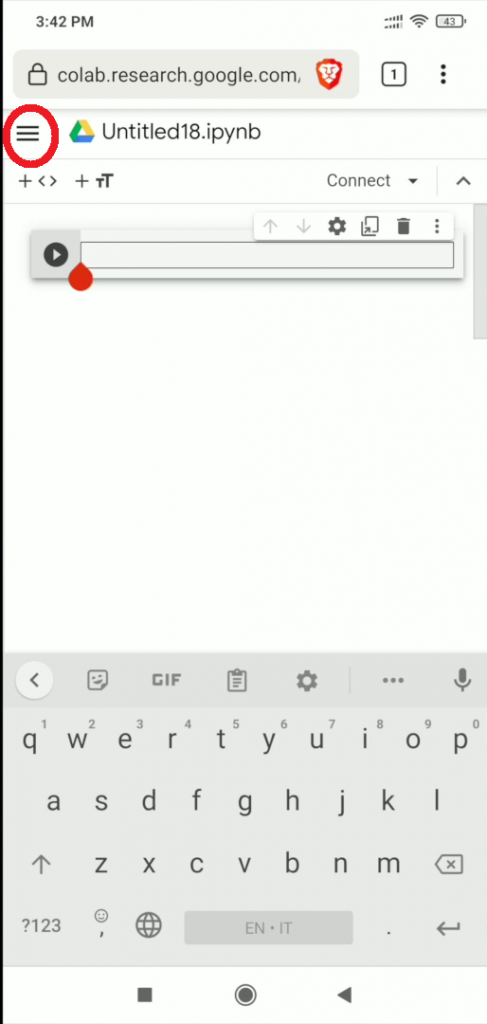**Detailed Caption:**

The image captures a screenshot from a mobile phone using the Brave browser, identified by the screen dimensions which are approximately three times as tall as they are wide. The screenshot was taken at 3:42 p.m., as indicated by the timestamp at the top. There are two sets of network reception indicators, suggesting the phone may have dual SIM capabilities, with one showing four bars and the other five bars of signal strength. The Wi-Fi signal is strong, and the battery level is at 43%.

Dominating the screen is a browser window with the URL partially visible: "colab.research.google.com". The user has annotated the screenshot by circling the three-bar hamburger menu icon and highlighting the Google Drive logo next to the label "Untitled 18.ipynb".

The main content area of the browser window is largely empty, except for a play icon next to an entirely empty progress bar, indicating a lack of loaded content or a paused operation. The lower portion of the screen, occupying about 25-30% of the display, shows the on-screen virtual keyboard, ready for the user to input text, presumably into a search box or form field.